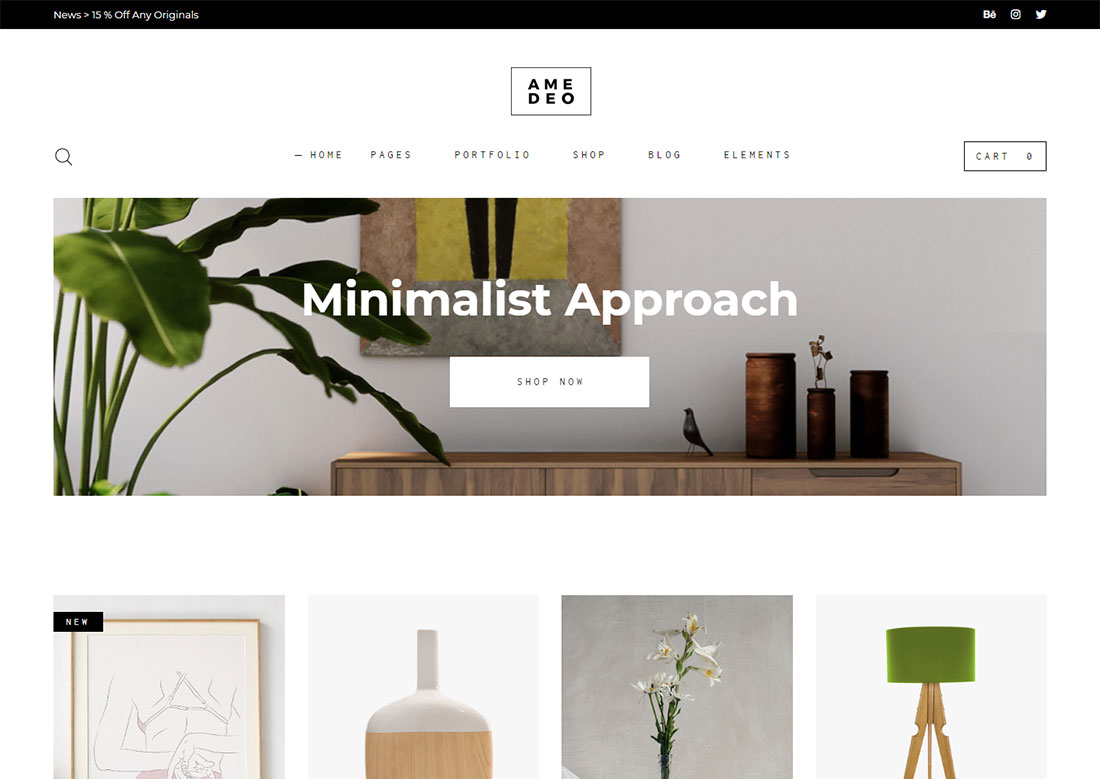The image depicts the front page of a modern, minimalistic online store. The top portion features a black banner stretching across the page, with "News: 15% off any originals" prominently displayed in white on the left. On the right side of this banner, there are white icons for Twitter and Instagram. Below this, the background is predominantly white. 

Centrally positioned under the banner is a black-outlined box with the text "A-M-E-D-E-O" inside. Below this, a large, rectangular photograph spans the width of the page. The left side of the picture showcases a plant with large green leaves extending towards the camera. A wooden table is partially visible in front of the plant, adorned with various vases and a small decorative black bird. Above this area, white text reads "Minimalistic Approach."

A "Shop Now" button is centrally placed beneath the text. To the right of the button, there is additional decor: a brown canister, a smaller canister with sprouting leaves, and another slightly larger canister. In the background, a gray wall hosts a painting's lower section, featuring a yellow backdrop and the black pant legs of a figure. 

Below this central image, four purchasable items are displayed: a sketch, a large moonshine jug with a white top and brown wooden sides, a green-stemmed plant with white and pink flowers, and a modern lamp with a green shade and wooden tripod legs.

The overall design is sleek and elegant, aligning with the store's minimalist theme, aimed at showcasing home accessories and modern decor items.